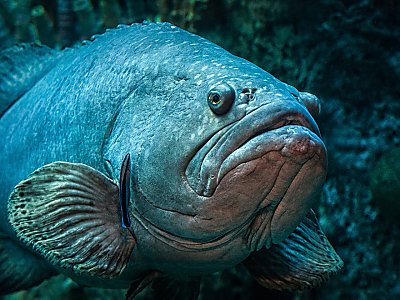This close-up image captures a very large, bluish-gray fish partially out of frame, facing to the right with an olive-shaped eye and a somewhat open, frowning mouth. The fish appears very fat and has two prominent fins in front, with a spiky top fin and part of a back fin visible. The background is slightly blurred, revealing greenish plants or possibly algae, and a dark rock. Though the water is not visible, being a fish suggests it is underwater. The setting is dark, with the fish being the central focus against a bluish and somewhat obscure environment.